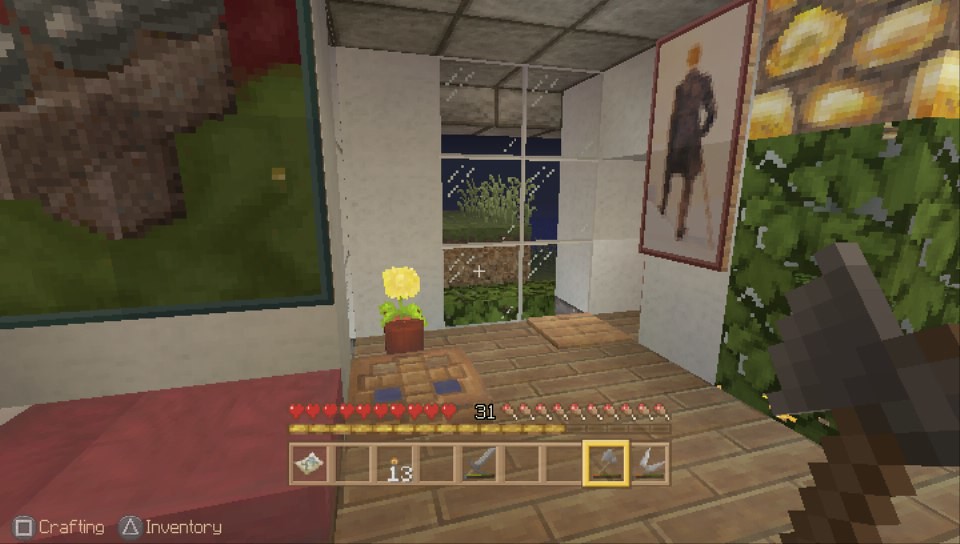This image is a low-quality photograph from a video game, resembling a scene from a platform like Second Life or Minecraft with a texture pack installed. We are inside a fairly modern-looking house with white walls and tan brick floors. Dominating the space in the rear center is a six-pane, floor-to-ceiling window looking out to what appears to be nighttime and some green plants or a hill with grass. The ceiling features rectangular off-white panels forming a drop ceiling.

On the right-hand side of the image hangs a wooden-framed portrait of a man in a black morning coat with a cane, while the upper right corner shows a brick stone wall with leafy patterns on the lower part. To the left is a red fabric piece, likely a bed, with a label in lighter letters reading "crafting and inventory." There's a large, dark green painting above it that seems to depict stone elements.

The bottom of the screen displays game interface elements: a row of nine icons indicating various game functions, such as switching objects and power levels, with a number 13 and some empty slots. Above this, on the left, is a series of red hearts indicating full health and on the right, flowers or similar objects with the character at level 31. Additionally, the inventory shows a map, 13 torches, stone tools, and other items, suggesting the player has practical supplies for exploration or building.